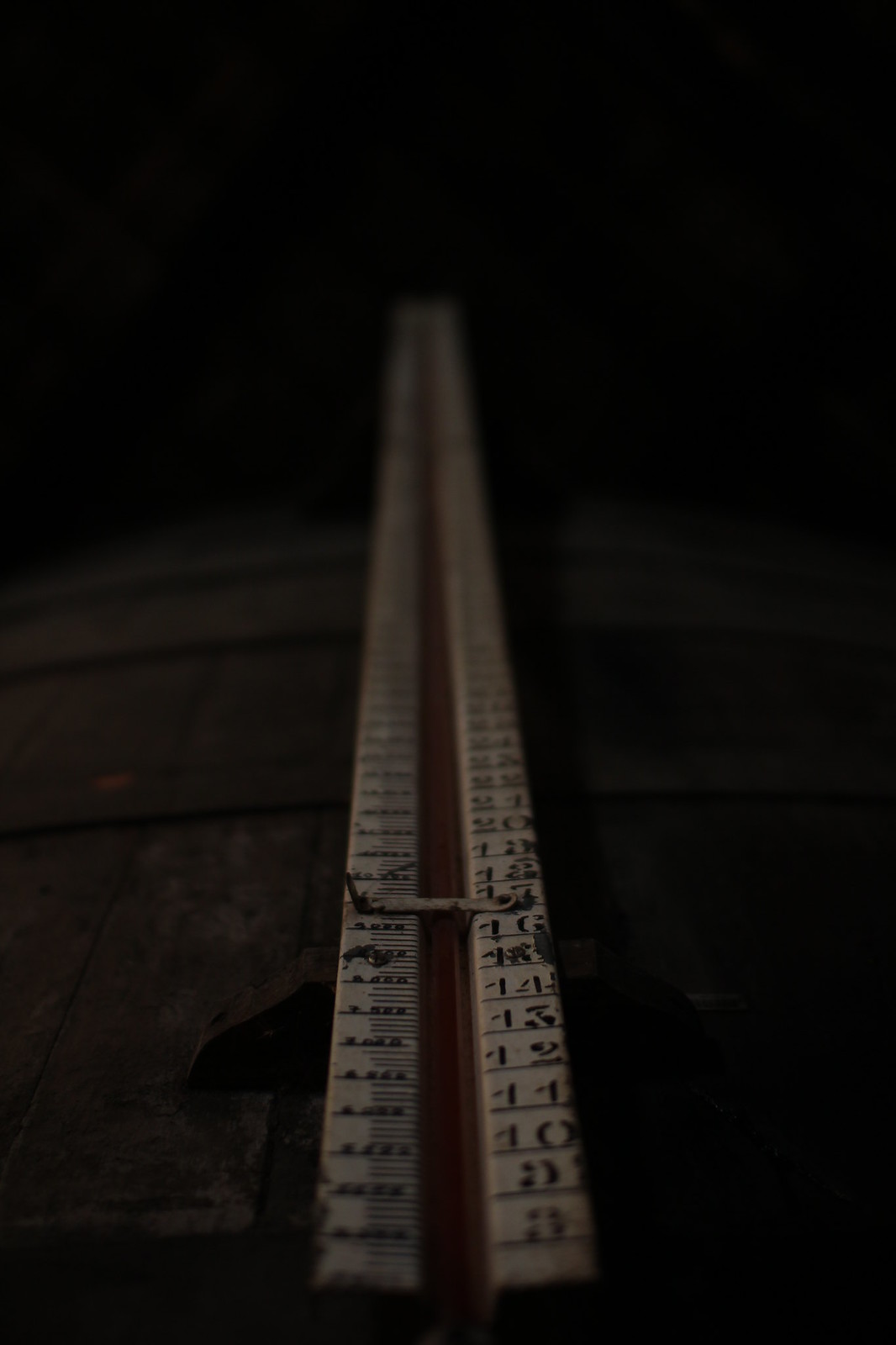This photorealistic image provides a close-up view of an elongated measuring device, prominently featured in the lower half of the composition where it is in sharp focus. The device comprises two lengthy white rods marked with various numbers and separated by a central red section. Approximately one-tenth of the way up from the bottom lies a metal slider, designed to move vertically along the rods to facilitate precise measurements. This particular measuring device is affixed to what appears to be a wooden barrel, identified by its clearly defined wooden slats. The connection is secured by a rusted, dark brown metal fastener. In the background, the wooden slats continue horizontally, gradually becoming more blurred and losing detail as they recede from the focal point. 

On the right rod of the device, large, clearly visible numbers range from 8 to 24, although the number 15 seems to be scratched out. Towards the left side, the numbers are notably smaller and interspersed with fine markings indicating more precise measurements. The overall image is dark, suggesting it was taken indoors under low lighting, capturing the texture and material details in a realistically gritty manner.